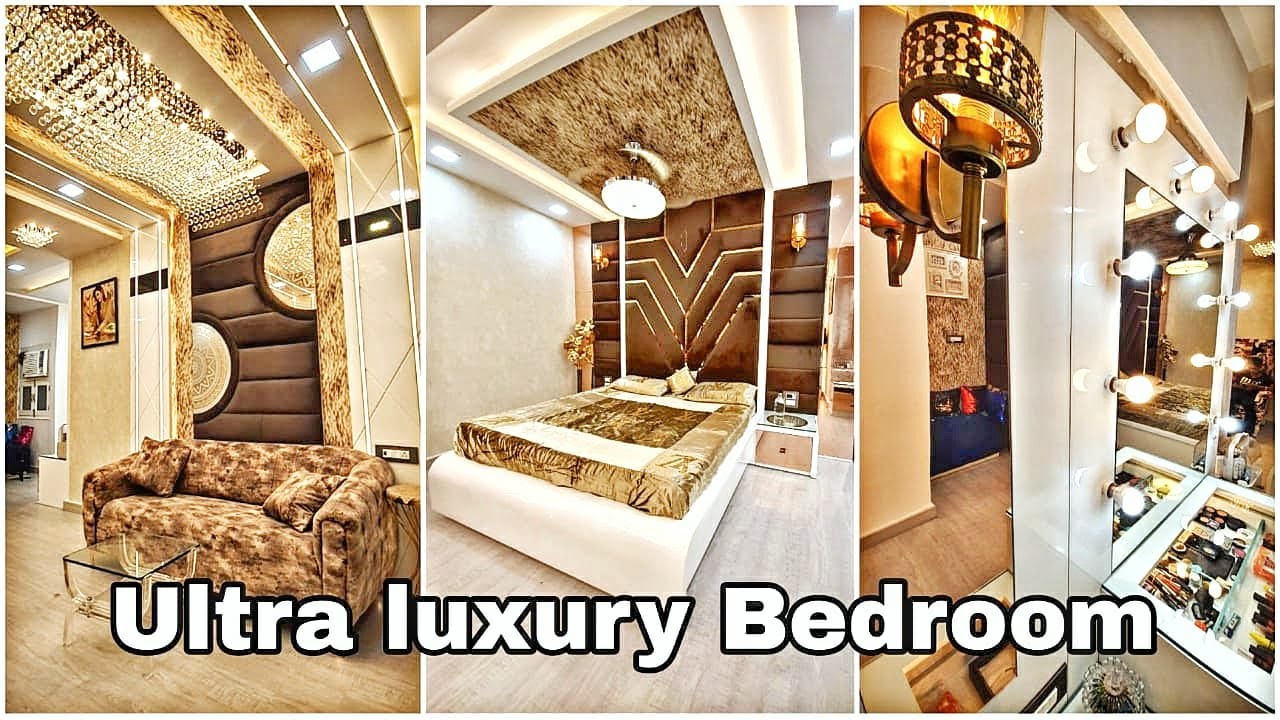This multi-panel image, captioned "Ultra Luxury Bedroom" in bold white outlined in black at the bottom, showcases three distinct interior shots emphasizing opulence and design intricacies. The leftmost panel features a stylish living area with a brown couch in front of a glass coffee table. The room is adorned with a wood-paneled wall, two decorative half-circle lights, ceiling lights, and a wavy strip of lighting accentuating a picture on the wall, all resting on a wood floor. Moving to the center panel, the focal point is an extravagant bed adorned with white and brown covers, resembling a bed over a bed due to the larger white portion and a smaller brown border. Above the bed hangs a unique, almost furry decorative chandelier, set against a backdrop of V-shaped wood panels and flanked by elegant lamps on either side. A wooden nightstand completes the setup. The rightmost panel presents a luxurious vanity area featuring a mirror surrounded by multiple traditional halogen lights, evoking a vintage Hollywood glamour. The reflection in the mirror hints at additional furnishings, possibly a blue chair, and beneath it lies a storage unit, possibly for makeup or other personal items. Each panel underscores the use of browns, golds, and beige tones to create a cohesive, luxurious atmosphere.